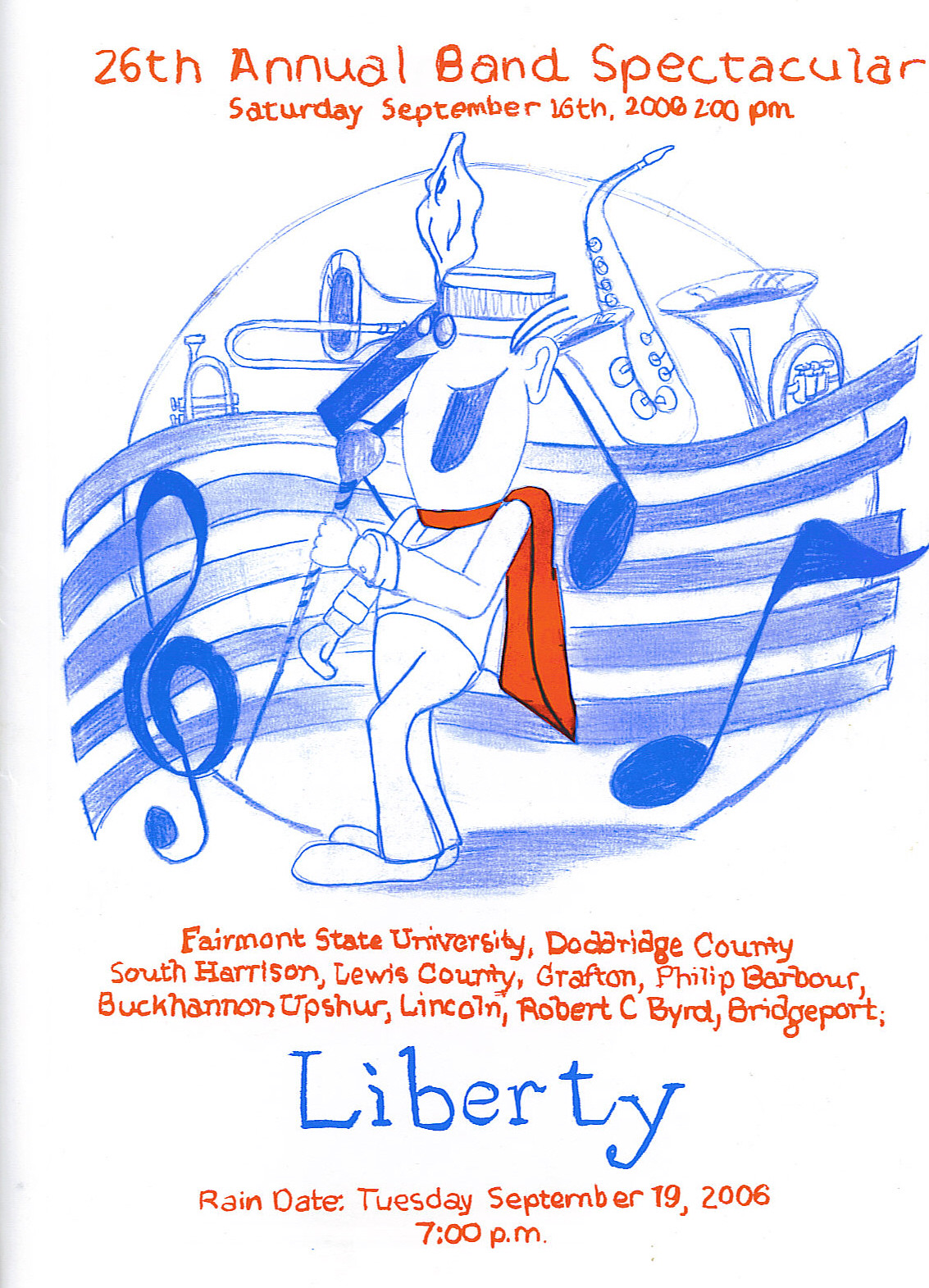The image is a detailed, hand-drawn poster advertising the "26th Annual Band Spectacular." The poster predominantly features red and blue hues on a white background, with red and blue lettering. In the center, a character, who appears to be a marching band leader, is illustrated in a cartoony yet detailed style using blue color pencil. The character is wearing a red scarf and a hat, and is depicted singing into a microphone with musical notes floating around him. Behind him are various wind instruments such as saxophones and tubas. The text at the top announces the event: "26th Annual Band Spectacular, Saturday, September 16th, 2006, 2 p.m." Below this, more information is provided in red letters: "Fairmont State University" followed by a list of counties including Doddridge County, South Harrison, Lewis County, Grafton, Phillip, Barbour, Buckhannon, Upshur, Lincoln, Robert C. Byrd, and Bridgeport, with "Liberty" uniquely highlighted in blue letters. The rain date for the event is also mentioned: "Tuesday, September 19th, 2006, 7 p.m." Overall, the poster's vibrant and illustrative style adds a personal touch to the event advertisement.